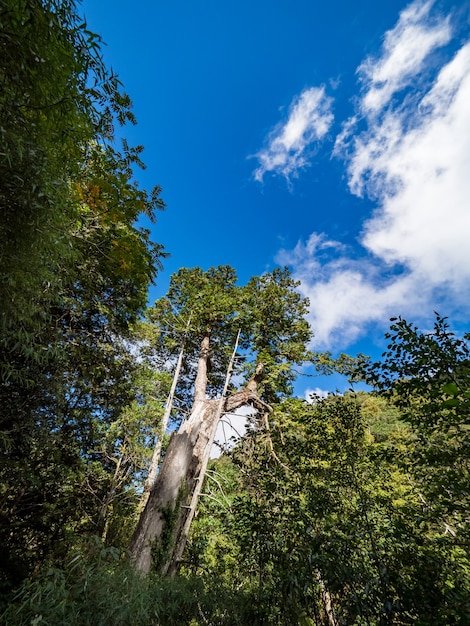The photograph captures a striking upward view from the base of a prominent beige-white tree trunk that splits into two thick branches, extending into a canopy of dark green leaves. Surrounding this central tree is a dense forest, with a variety of trees of different heights and trunk sizes, their foliage lush and verdant. The scene is framed by a vibrant blue sky scattered with a few thick, white clouds, particularly visible in the top right corner. On the top left, additional trees are visible, filling the frame with greenery. In the background, a greenish hill cloaked in foliage adds depth to the image, enhancing the natural beauty of the scene.